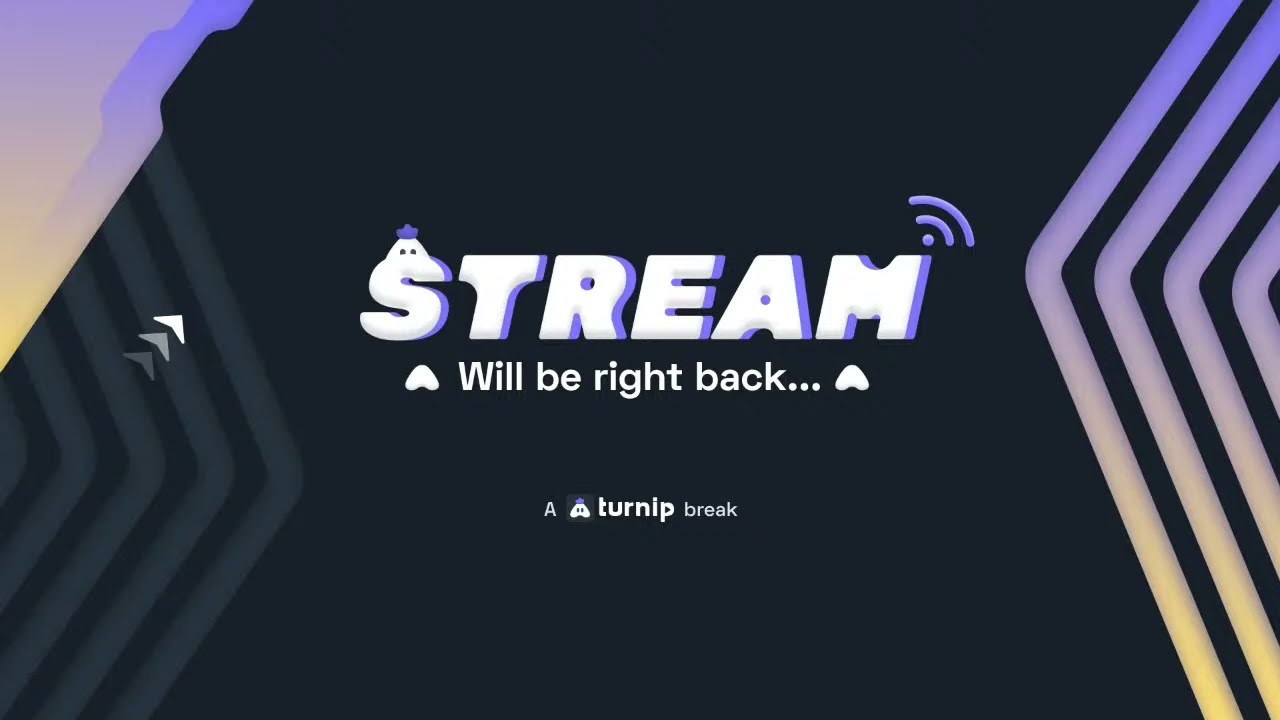This image is a piece of clip art or a poster ad with a primarily black background. In the center, the word "STREAM" is prominently displayed in white font with a light purple or lavender drop shadow behind the letters. Above the "M," there is a small Wi-Fi icon, akin to the signal indicator on a phone. Below "STREAM," the text "We'll be right back..." is written in white font, followed by the phrase "A Turnip Break," with "TURNIP" bolded. Various triangular shapes resembling boomerangs or game controller icons accentuate the design. On the left, dark charcoal triangles point towards the center, while on the right, light purple triangles transitioning to yellow create symmetry. Additionally, an odd little creature-like icon appears next to the word "TURNIP" and atop the "S" in "STREAM." The corners of the image feature angled triangular designs, with the top left corner displaying a flattened thick border shaded slightly pink. The right side has purple and yellow triangular shapes that angle outward, creating a dynamic border effect that fades from orange to blue on either side of the slide.